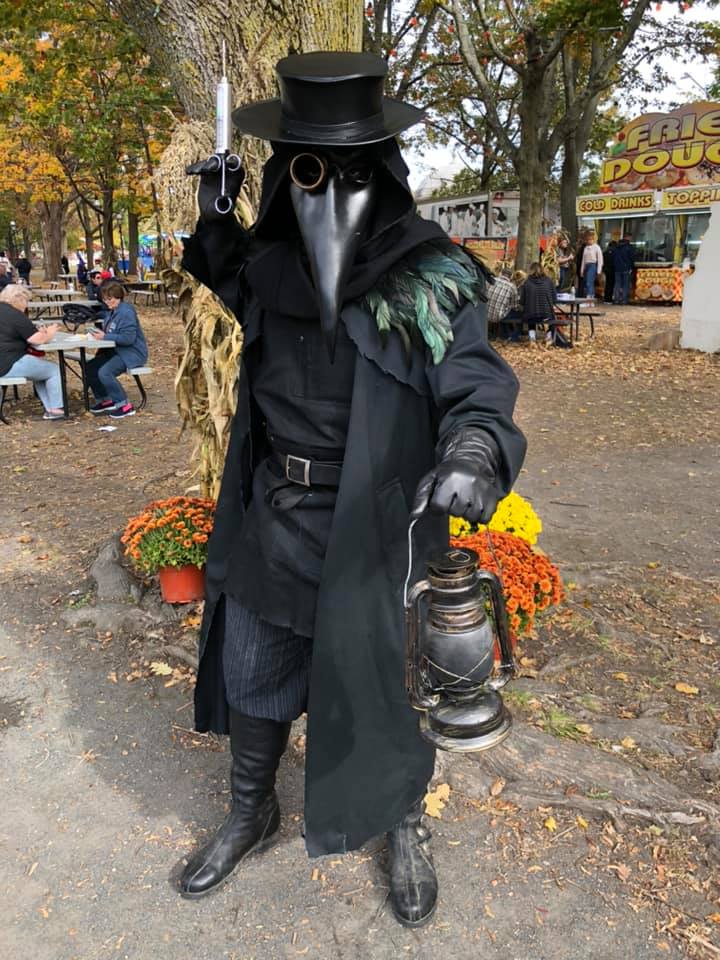In this captivating outdoor photograph, a mysterious figure dressed head-to-toe in an elaborate plague doctor costume commands attention. The costume features the iconic long-nosed mask with goggles, adorned with feathers on their shoulders, and they wear a flat-brimmed black top hat. The outfit includes a long black trench coat, billowy pants, and tight black boots, completed with leather gloves. The individual holds a black kerosene lantern in their extended left hand and an old-style silver surgical syringe in their right hand, brandishing it prominently.

The setting, likely a fall or Halloween festival, is colorful and bustling with activity. The person stands on what appears to be a street or a courtyard with a decorative tree nearby, surrounded by yellow and orange mums. In the background, a food truck or stand labeled "Fried Dough" is visible, indicating a festive, fair-like atmosphere. Numerous individuals not in costume are seated at picnic tables, eating and chatting, enhancing the vibrant sense of community and celebration in the autumnal outdoor setting.